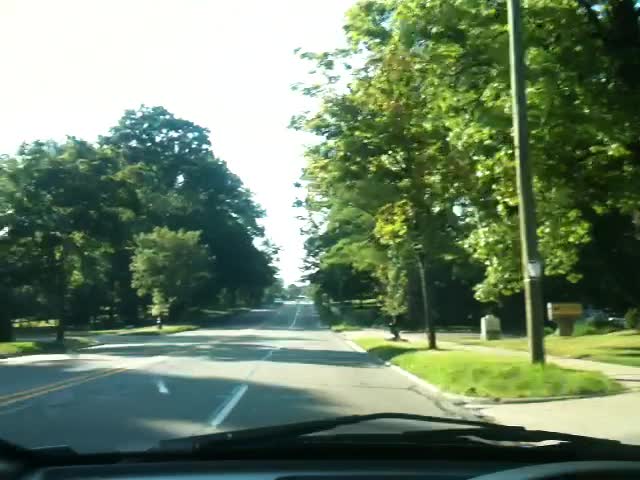The photograph, taken during daylight from inside a vehicle, offers a partial glimpse of the car's dashboard along with black windshield wipers. The scene captures a road with light gray pavement, marked by a white strip running down its center and yellow lines off to one side. The road is flanked by lush, bushy green trees and a lighter green expanse of grass. A light pole is also visible, standing along the tree-lined street. A sidewalk runs parallel to the road, bordered by grass that reflects shadows of tree branches and leaves. The image quality is decent but slightly grainy, and a portion of the sky can be seen overhead.